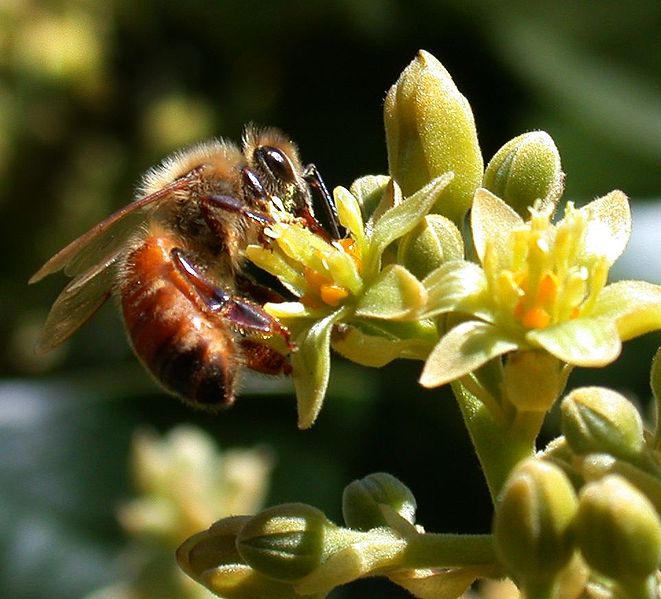This is a stunning, professional close-up photograph capturing a bee in remarkable detail as it gathers nectar from a newly opened yellow flower. The bee, situated on the left side of the image, is the star of the composition. Its large, expressive brown eyes and the delicate tan hairs on its body are illuminated by sunlight, creating a glowing effect. The translucent wings reveal a hint of the blurred green background through them, adding to the ethereal quality of the scene.

The right side of the photo showcases the flower in intimate detail. The yellow bloom is surrounded by buds mostly still closed, with pestles projecting little orange spots of nectar, eagerly awaited by the bee. The plant itself, likely from a garden, exhibits a vivid contrast between its green stems and the bright yellow flowers. The overall background is a soft blur of green, keeping the focus squarely on the intricate interaction between the bee and the flower. This composition, devoid of any text or human presence, truly highlights the delicate and beautiful moment of pollination in nature.